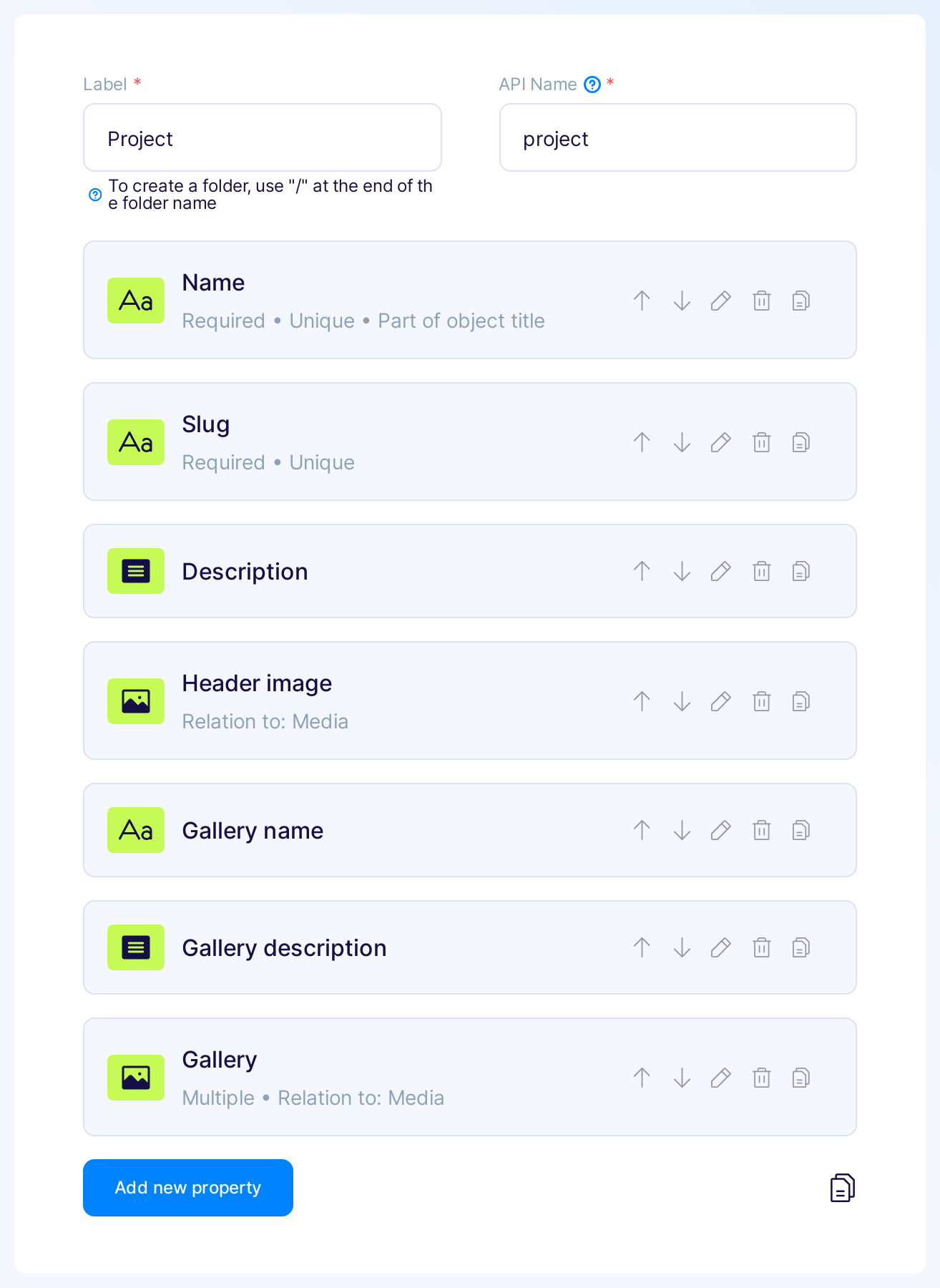The image features a detailed interface layout, likely from a software or web application. 

In the top-left corner, there's a label followed by a star icon, indicating a required field. Below this label, a rectangular section displays the text "Project API Name" accompanied by a question mark and a star icon, possibly suggesting that additional information is required. 

Beneath this heading, there is another rectangular box containing an input field with placeholder text that reads "Project." The field is designed for entering a project name. Adjacent to this input field is a text label with the letter "A," providing further instruction or annotation. The text "Name, required, unique" is also visible, implying that the name must be unique and is a mandatory field. Next to these instructions, there is an icon of a pen (for editing) and a trash can (for deletion).

Further down the interface, similar elements are repeated for the "Slug" field, marked as "required" and "unique." This section, too, is accompanied by the pen and trash can icons for editing and deleting, respectively.

Below these fields, there's a segment labeled "Description," which presumably expects a brief summary or explanation related to the project.

Towards the lower part of the image, the word "Gallery" is displayed, possibly indicating an area related to media or image uploads. There is also a mention of "Property," which might refer to individual gallery items or attributes.

To the right, there is a visual depiction of various items or entries, described as blue circles with unspecified properties against a white background. The entire layout suggests a well-structured form for inputting detailed project information within a software or web application interface.